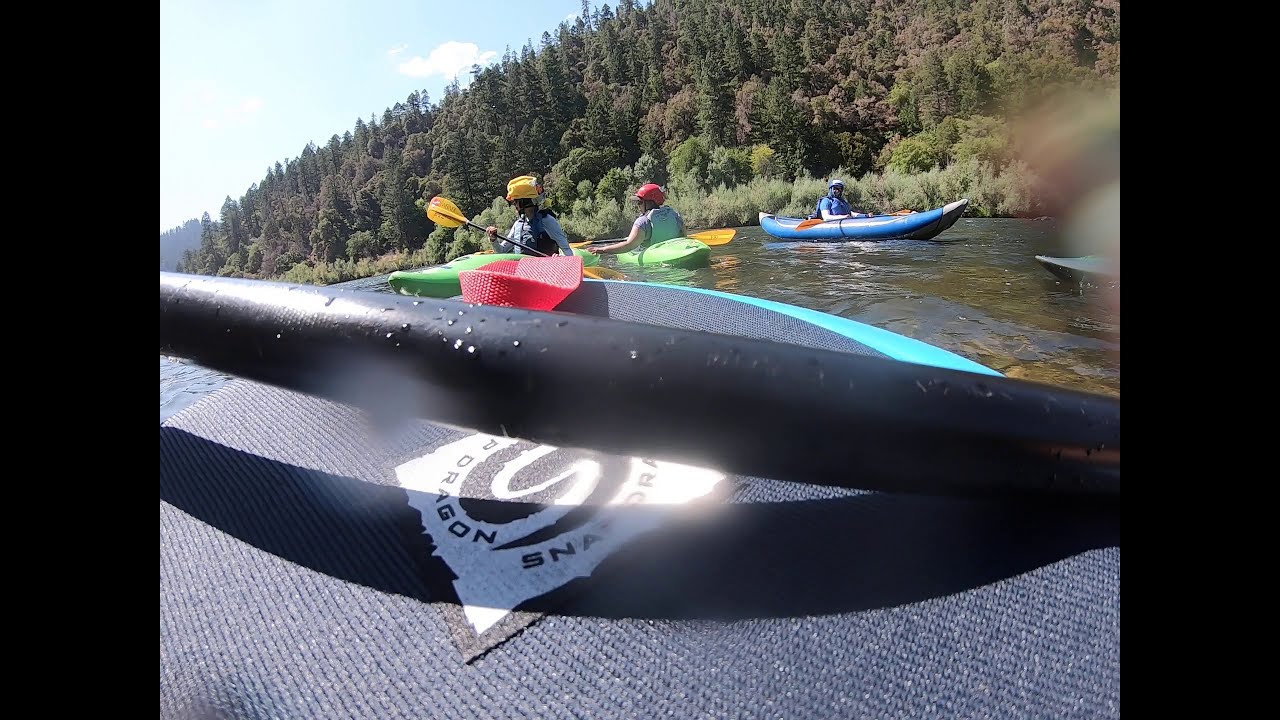In this vibrant image, taken from the vantage point of a kayaker, the foreground features the nose of a turquoise kayak adorned with an S-shaped logo, and a black paddle crossing the middle of the screen. The scene is set on a serene river, its greenish water reflecting the mid-day sun. The backdrop is a lush expanse of evergreen trees covering a hill or mountain, evoking the landscapes typical of the northwestern United States. In the water, four kayakers navigate their colorful vessels: two in green kayaks, one in a blue kayak, and the photographer's turquoise kayak. The kayakers are easily distinguishable by their helmets – one yellow, one red, and one blue – adding a splash of color to the scenic natural setting. The water is calm, enhancing the peaceful and adventurous atmosphere of the scene.